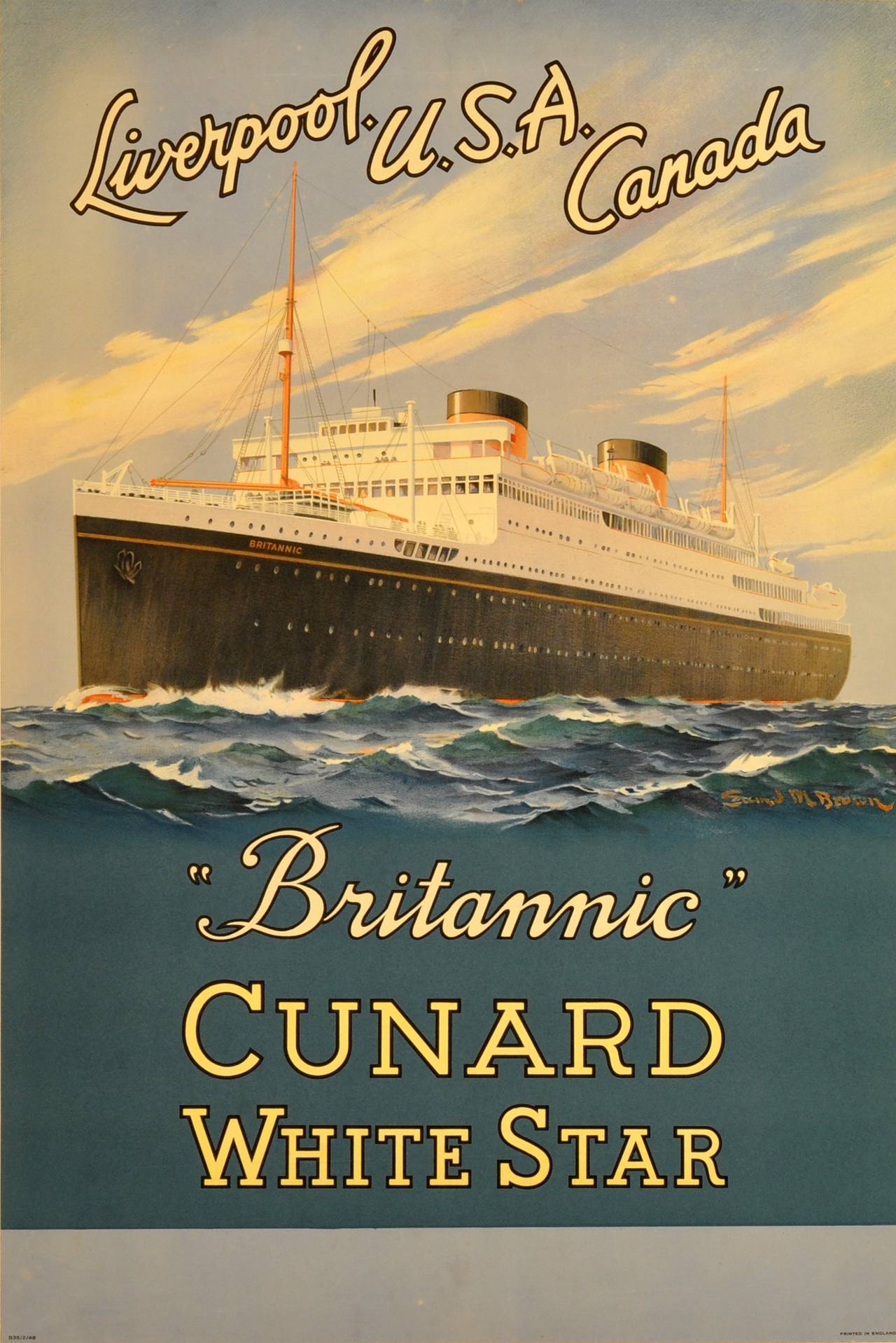This vintage advertisement features a beautifully painted illustration of the Britannic, a cruise liner from the Cunard White Star line, prominently showcasing its destinations: Liverpool, USA, and Canada. The central image is a detailed depiction of the ship itself, rendered in a style reminiscent of the 1950s or 1960s, reflecting the artistic aesthetics of that era. The Britannic is seen sailing through slightly choppy blue waters under a clear blue sky adorned with three wisps of clouds. The ship boasts a wide base, a black hull with a distinctive yellow stripe in the middle, and a white upper deck, topped with two prominent stacks. Text in an italic script frames the composition: "Liverpool, USA, Canada" is displayed at the top, while "Britannic" in quotes, followed by "Cunard White Star" in yellow type with a black border, is positioned below the ship. The artist's watermark is subtly incorporated within the water, adding a unique touch to the piece.